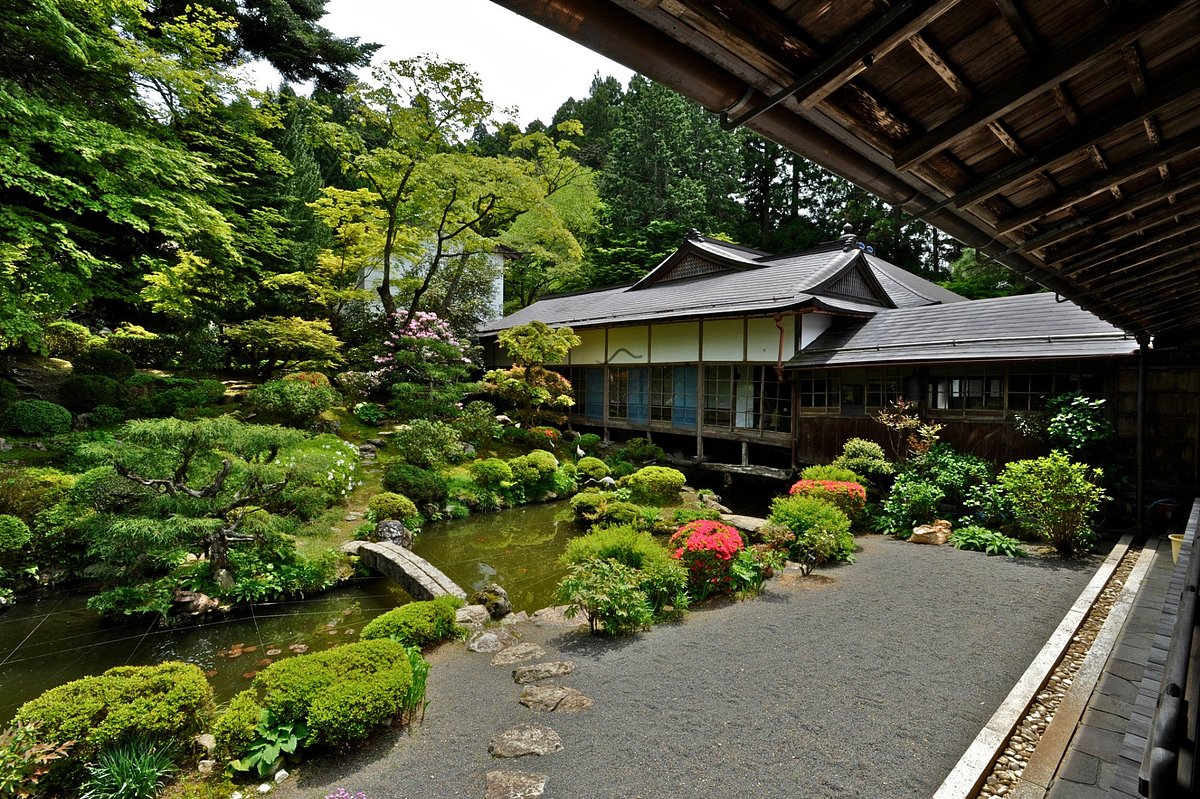This vibrant photograph captures a serene scene from beneath a wooden awning attached to a traditional Japanese-style building with steep, decorative rooftops. The image showcases a lush garden, featuring a rich tapestry of green bushes, trees, and various thoughtfully planted shrubs. Accents of pink, red, and orange flowers add splashes of color among the foliage. A small, graceful stream or pond flows through the scene, spanned by a quaint stone bridge that leads from a rock-strewn path to an inviting garden. Tall, slender trees with splayed leaves thrive in this meticulously landscaped oasis, creating a sense of tranquility and harmony. The backdrop is a white-walled structure embodying traditional Japanese architecture, enhancing the overall impression of an idyllic, well-maintained garden retreat.